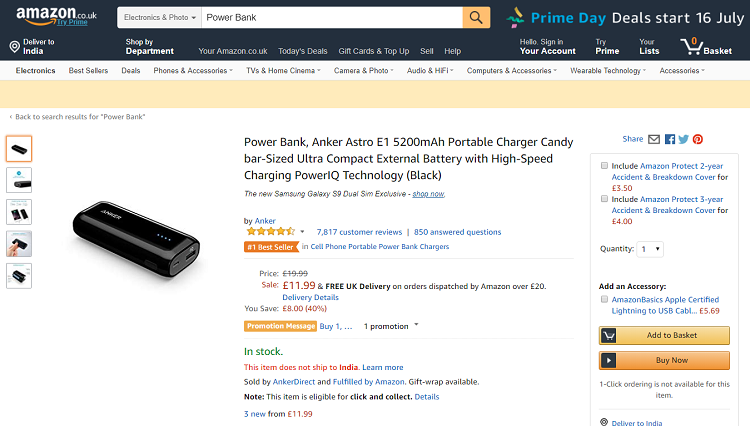This is a detailed screenshot taken from the UK Amazon site. At the top left, there is a note indicating delivery to India. The shopping basket is currently empty, and the user has searched for "power bank" under the electronics and photo filter section. The primary item displayed is a black power bank from the brand Anker, spelled A-N-K-E-R. On the left side of the screen, there are five smaller images that allow for zooming in to view specific details of the product. The main image on the right showcases the sleek design of the Anker power bank. The customer reviews accompany the item, and it is priced at £11.99, discounted from the original price of £19.99. The product is noted as being in stock but has not been added to the cart. Additionally, there is a promotion message mentioned which hasn't been accessed yet. The listing indicates that the product is sold by Anker Direct and fulfilled by Amazon.